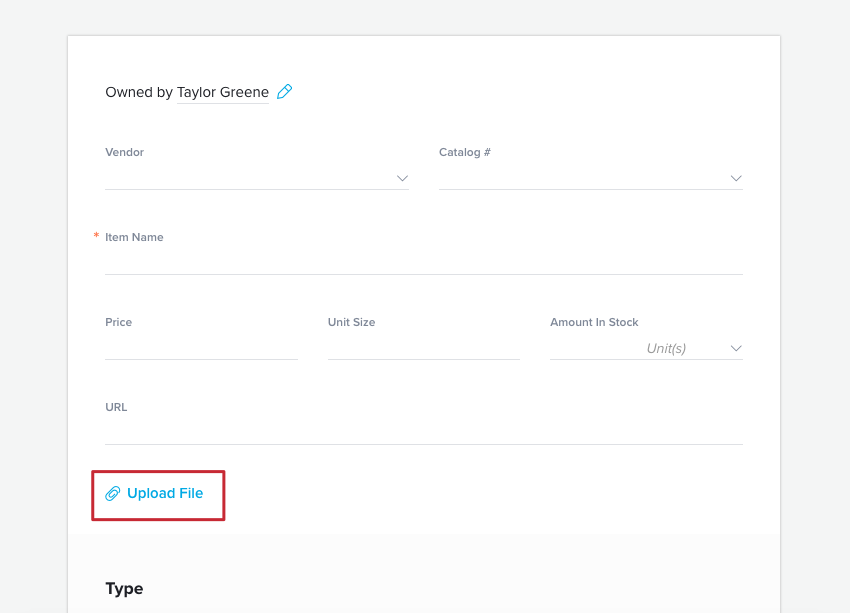The image is a screenshot depicting a blank text document with a white background and a light grey border, partially visible, suggesting either it is the first page or further scrolling is necessary to view its entirety. At the top, there is a title stating "Owned by Taylor Greene" (Greene spelled G-R-E-E-N-E), accompanied by a small blue pencil icon designated for editing the title. Below the title, there are several lines and fields outlined in light grey for users to fill in information such as vendor, catalog number, item name, price, unit size, amount in stock, and URL. Additionally, a paperclip icon is visible with blue text that reads "upload file," which is prominently highlighted with a red box, indicating the uploader function's importance and drawing attention to it.